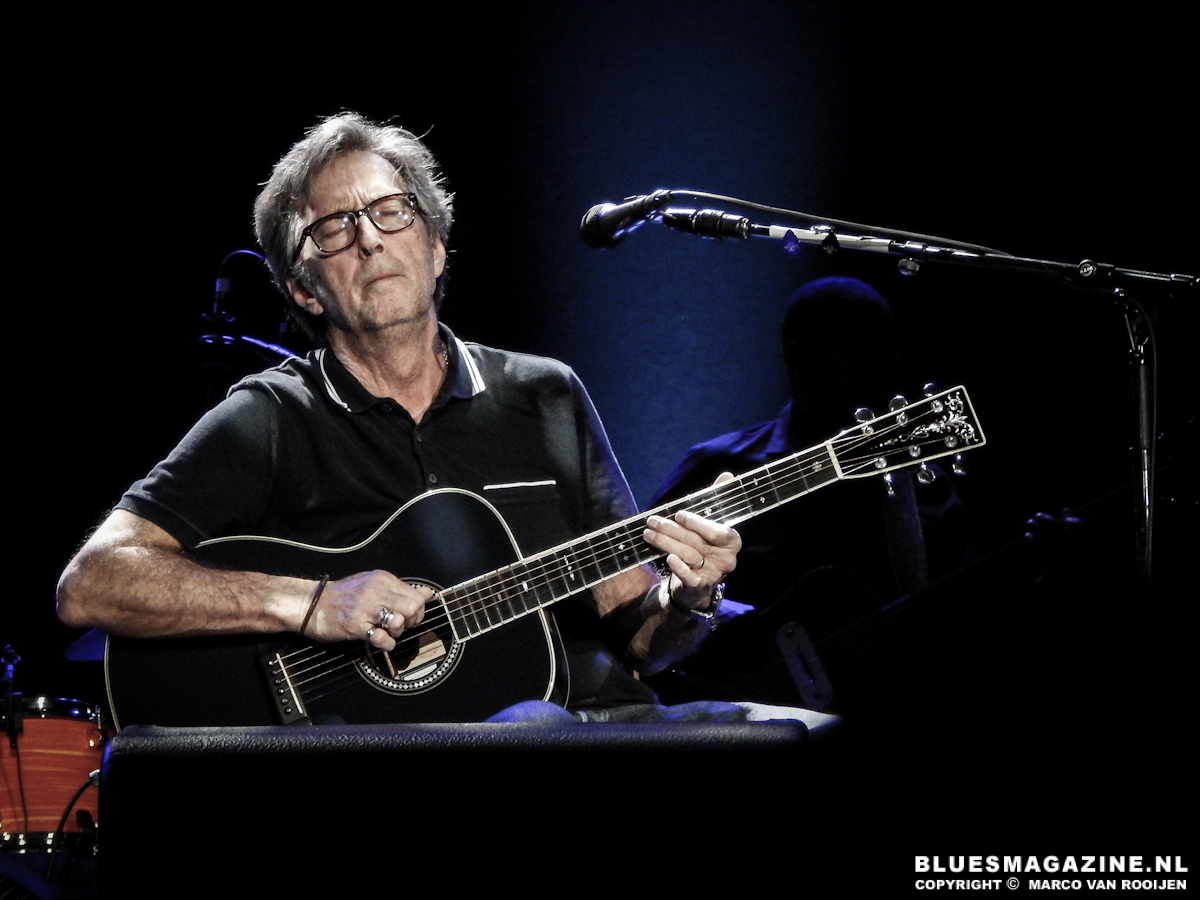The image features the renowned Caucasian guitarist and music artist Eric Clapton performing on a stage. Clapton, recognizable by his gray hair and glasses, is wearing a black polo shirt with a white pocket, with a collar that is black and white. In front of him is a black microphone with a stand, positioned close to his face. Clapton is intensely focused, eyes closed, as he strums a black acoustic guitar with some white detailing. The background is dark, but the blue lighting highlights Clapton and faintly illuminates another musician with short hair in the shadows behind him. On the bottom right of the image, "bluesmagazine.nl copyright Marco Van Rooijen" is prominently displayed. The scene is complemented by the presence of a brown drum and the plastic of an amplifier, situating Clapton mid-performance in what appears to be a recording studio or live music venue.